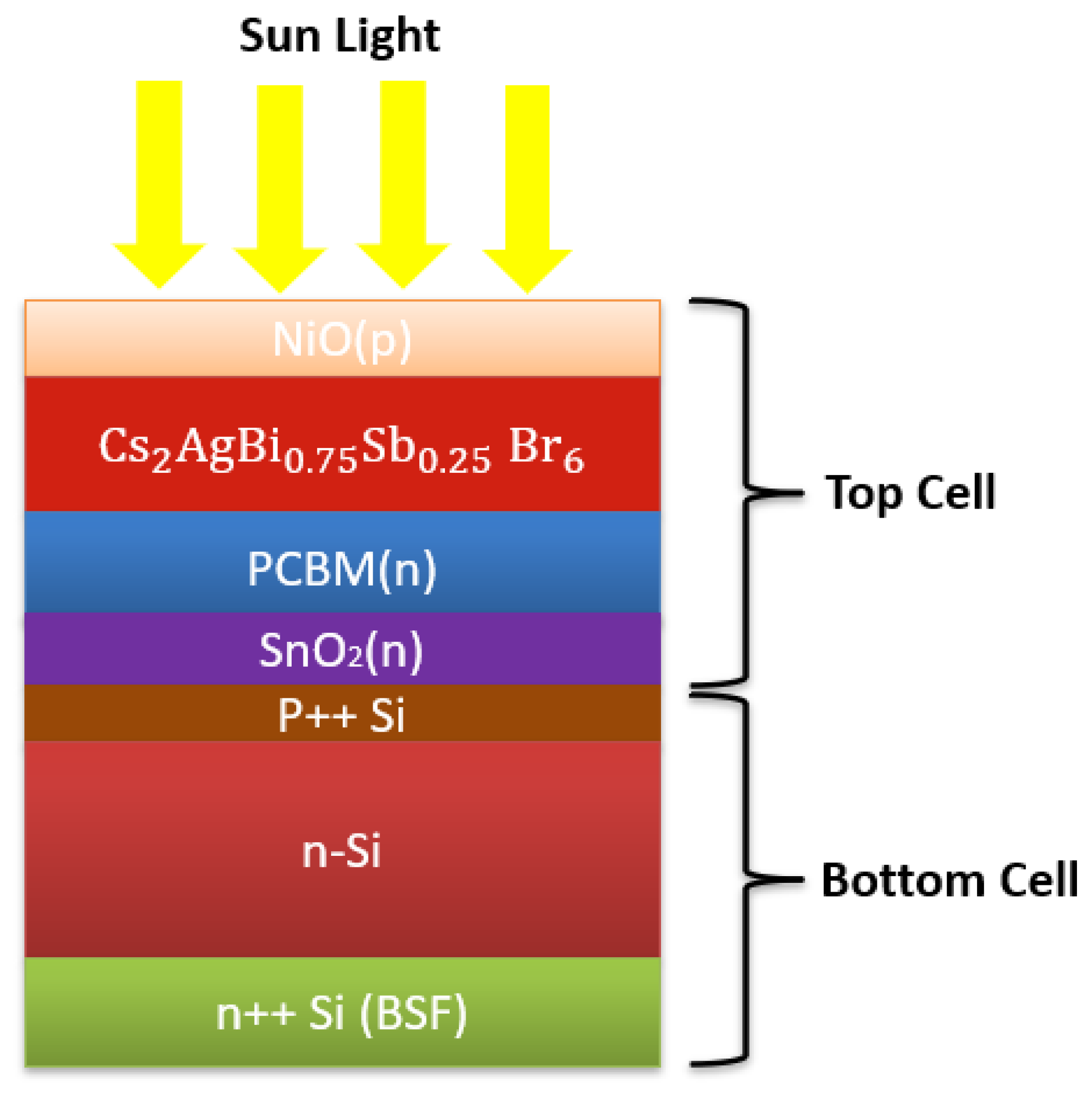The image is a detailed scientific diagram, likely relating to solar cells or a device that interacts with sunlight, presented in a somewhat cartoonish style on a white background. At the very top, it states "Sunlight" in black text, followed by four large yellow arrows pointing downward. Below the arrows, a horizontal rectangular graph is segmented into various colored horizontal strips, each symbolizing different materials or layers.

The first strip from the top is a creamish-tan color labeled "NIO (P)." The second strip is a burnt orange color, marked with the chemical equation "CS2ABAGBI0.75, SB0.25, BR6." The third strip is a light blue color, labeled "BCPCBM (N)," followed by a purple strip labeled "SN02 (N)." Sequentially, the fifth strip is brown and reads "P++SI," followed by another line in brown marked "N-SI," and the final green strip at the bottom is labeled "N++SI (BSF)."

On the right side of the graph, two black brackets are partially connected. The top bracket is labeled "Top Cell," encompassing the NIO (P), CS2ABAGBI0.75, SB0.25, BR6, BCPCBM (N), and SN02 (N) sections. The bottom bracket is labeled "Bottom Cell," covering the P++SI, N-SI, and N++SI (BSF) sections. This diagram likely explains the layered structure and chemical composition of a specific type of solar or electronic cell, demonstrated through varied color hues and detailed chemical formuli.